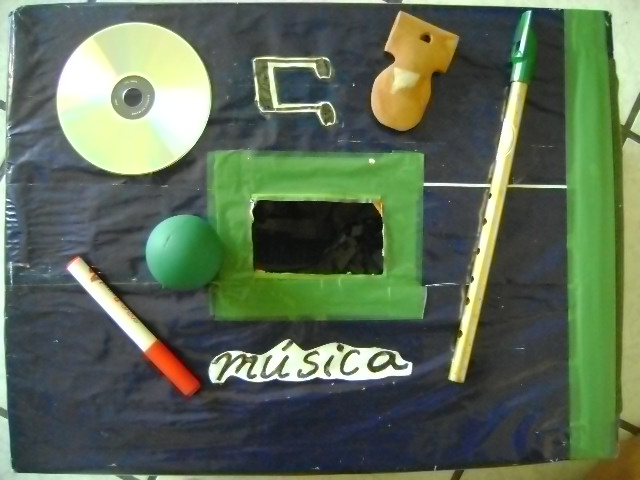This intricate artwork presents a multifaceted collage against a dark navy blue background. Dominating the image is the word "Musica," written in black marker on a piece of white paper that has been meticulously cut around its cloud-like outline. Positioned at the top left corner is a face-down silvery CD. Adjacent to the CD is a sideways musical note, also cut out of white paper and inscribed in black marker. 

Displayed along the right edge of the canvas is a bright Kelly Green strip. Intricately placed beneath it is a rectangular element with a green top and holes—possibly representing a handmade flute or recorder in a light cream hue. A peculiar, unidentifiable wooden object with a square top and a circular bottom rests nearby.

Below "Musica" on the left, a white pen with a red cap lies at an angle. To the left of this pen, near the center, is a small green ball set against another green square, enhancing the collage's texture. Completing the mixed media texture is a subtle strip of white tiles with dark brown grout, positioned as a backdrop behind the central elements.

This image is a rich combination of painted surfaces, cutouts, and everyday objects, harmoniously brought together to form a cohesive and engaging artistic composition.